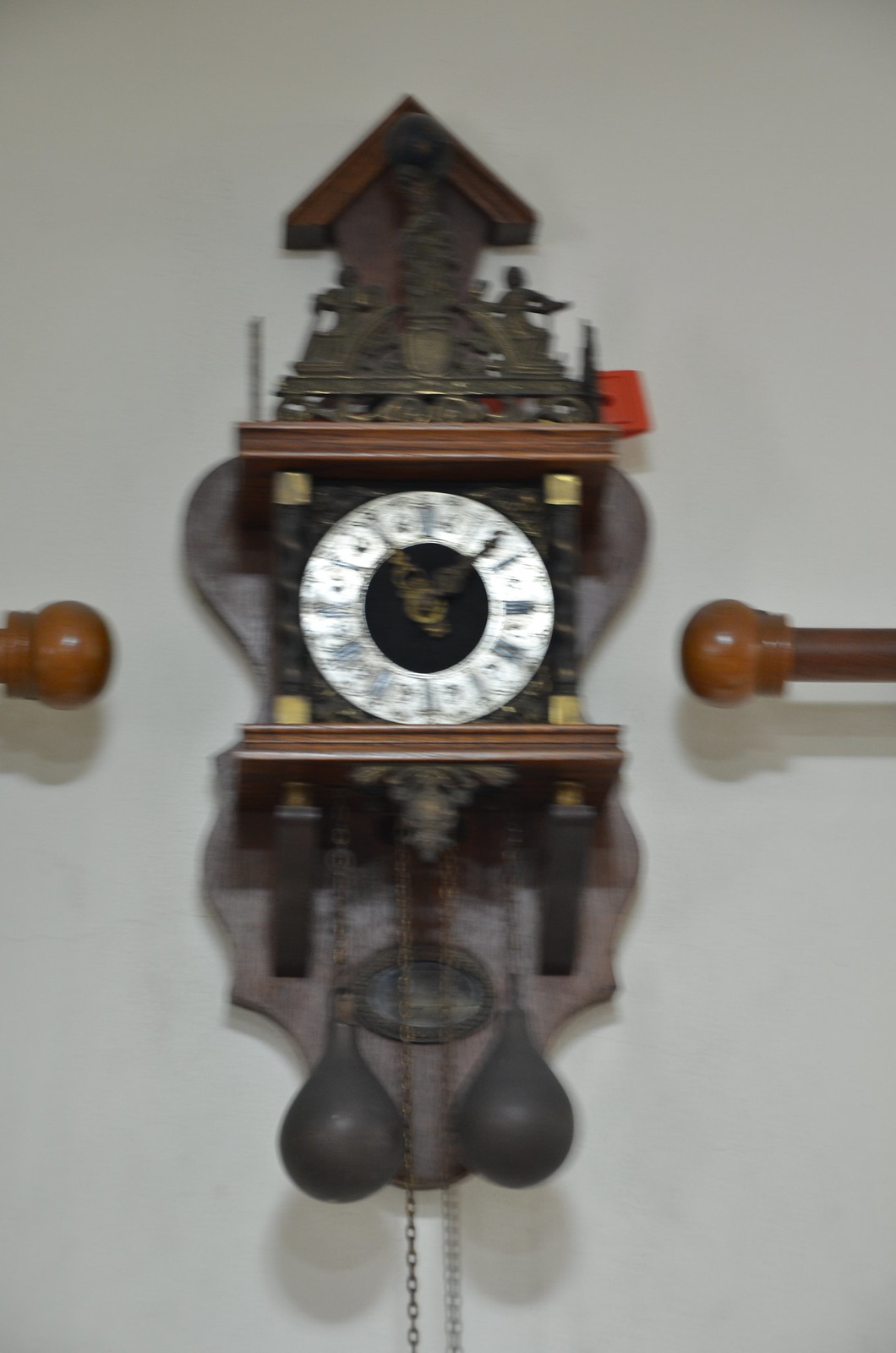This slightly out-of-focus photograph captures a detailed close-up of a tall cuckoo clock mounted on a wooden plaque, hanging on a white wall. The clock is positioned between two wooden curtain rods adorned with rounded finials at their ends, visible along the center-right of the image. 

The cuckoo clock itself features an intricate design, topped by a metallic scene depicting people, beneath a small angled wooden roof that is flush with the wall. The center of the clock has a black background with a white face showcasing Roman numerals. Elegant gold hour and minute hands mark the time, while four gold square accents adorn the top left, top right, bottom left, and bottom right of the clock face. A wooden border frames the top and bottom of the clock face, adding to its classic charm.

Beneath the clock face, two punching bag-shaped pendulums dangle from gold chains, with an additional two gold chains extending downward from their centers. The wooden plaque housing the clock is uniquely shaped, widening at the top, tapering in the middle, and ending in a rounded, pointed bottom. This detailed and intricate cuckoo clock serves as a beautiful focal point against the stark white background of the wall.